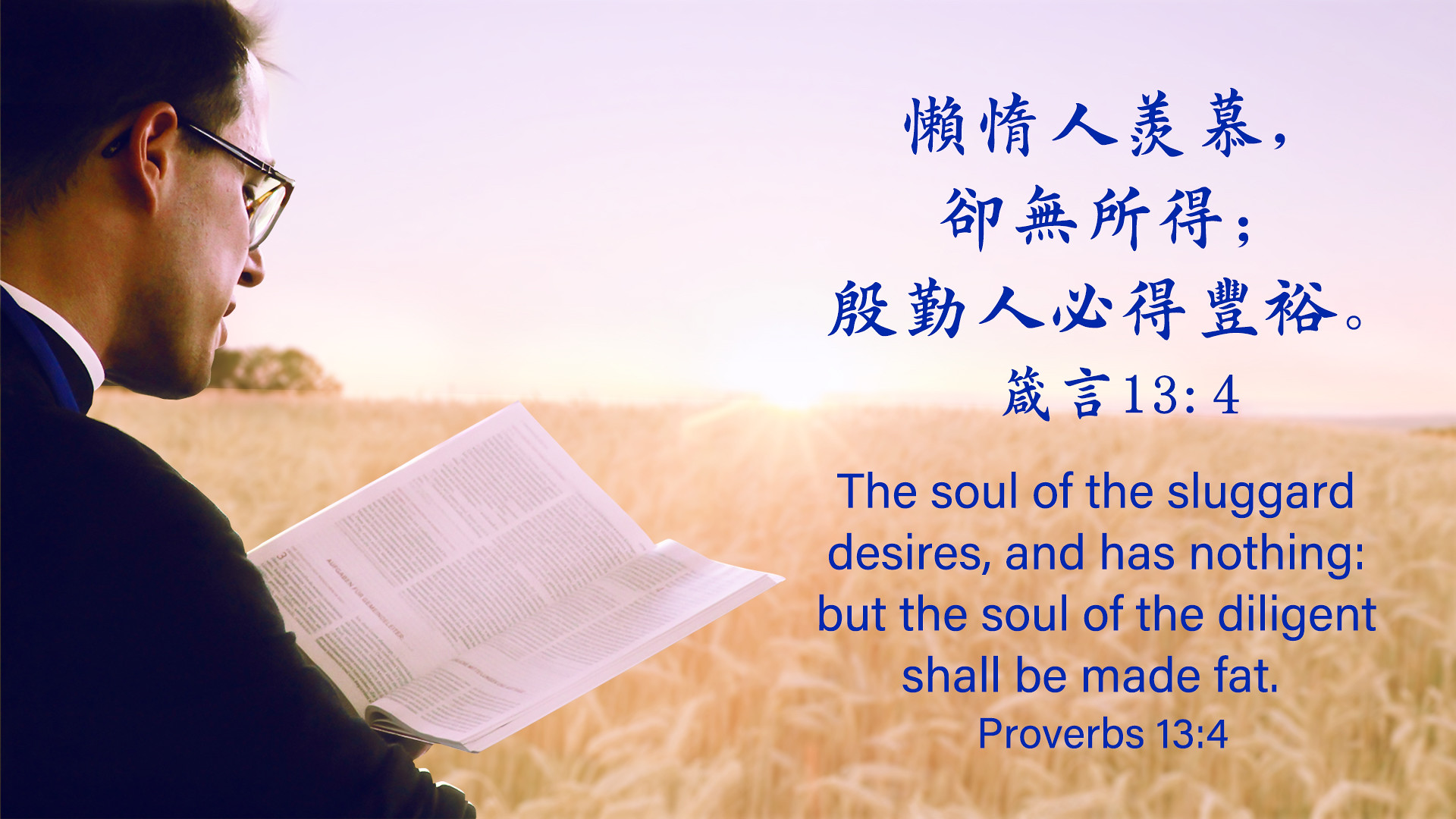This image is a religious graphic, possibly used for a church website, social media, or a sermon presentation. It features a young man, presumably a pastor, standing in a field that resembles a wheat or cornfield with the sunrise in the background. He is wearing a traditional black clerical robe with a white collar and a blue lanyard around his neck. Glasses adorn his dark brown hair, and he is holding and reading a booklet, likely the Bible. The man's right shoulder and back face the camera, leaving his front unseen. To the right of him, there is text, with a portion in either Japanese or Chinese characters in blue, followed by an English translation: “The soul of the sluggard desires and has nothing, but the soul of the diligent shall be made fat. Proverbs 13:4.” The background behind the text appears to be a grassy area, enhancing the overall serene and contemplative atmosphere of the image.